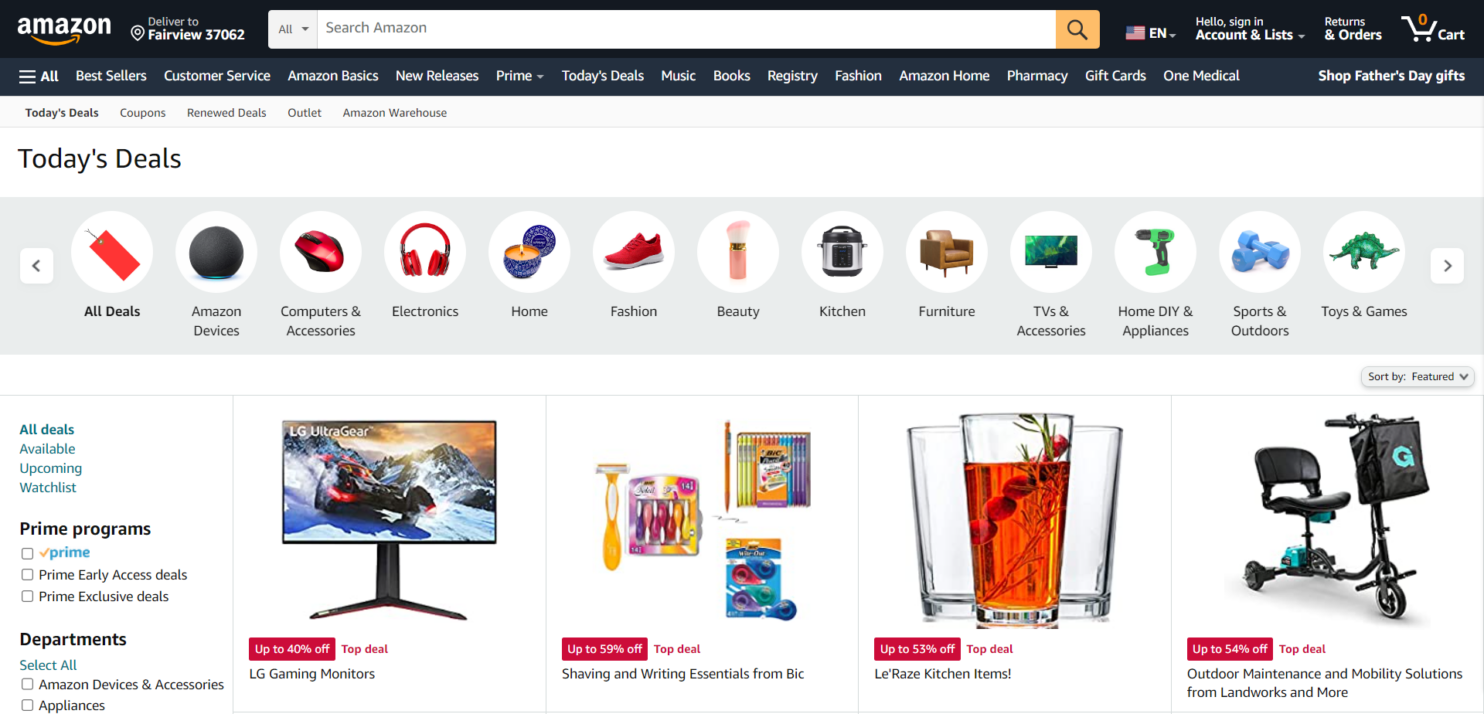This image captures a screenshot of the Amazon homepage showcasing daily deals. At the top of the screen, the delivery location is set to Fairview, zip code 37062, and the interface is in English. The search bar remains empty, indicating no current search queries. No user is signed in, and the cart is empty.

Dominating the screen is the title "Today's Deals," under which there are 13 categorized offers, navigable with right and left arrows hinting at more categories outside the visible area. The first four visible categories include: 
1. LG Gaming Monitors
2. Shaving and Writing Essentials from Bic
3. Kitchen Items
4. Outdoor Maintenance and Mobility Solutions from Landworx and others

Each of these categories is accompanied by corresponding images.

On the left side of the screen, there's a vertical sidebar labeled "All Deals," also organizing options such as "Available," "Upcoming," and "Watch List." Another section below lists different Prime Programs: Prime Early Access Deals, Prime Exclusive Deals, with none currently selected. Further down, under the "Departments" heading, there's an option to "Select All" highlighted in blue, with "Amazon Devices and Accessories" and "Appliances" listed underneath in black text.